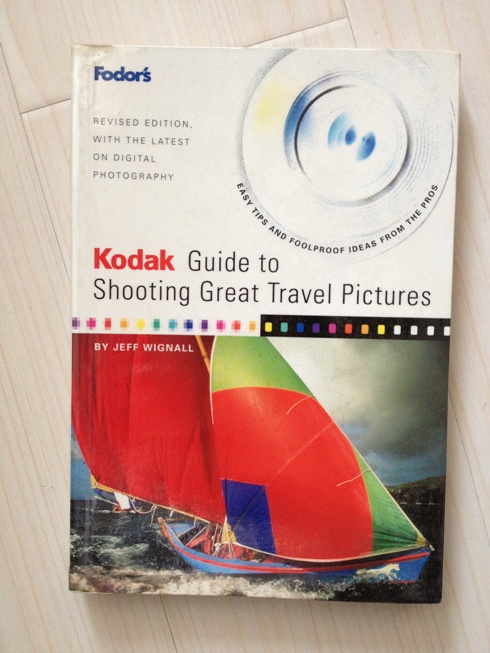This image depicts the cover of a book titled "Kodak Guide to Shooting Great Travel Pictures." The top half of the cover is predominantly white, featuring the text "Photos Revised Edition with the latest on digital photography." Additionally, it includes a small camera lens illustration in the top right corner, accompanied by the phrase "Easy tips and foolproof ideas from the pros." The central portion of the cover prominently displays the book's title and is attributed to author Jeff Wignall. Below the title, there is a dynamic photograph of a sailboat with vibrant sails in red, green, and blue, sailing on choppy water under a dark, cloudy sky. The sailboat itself is light blue with a red stripe. Above this image, a series of colorful squares are arranged in various hues, adding a splash of color to the overall design.